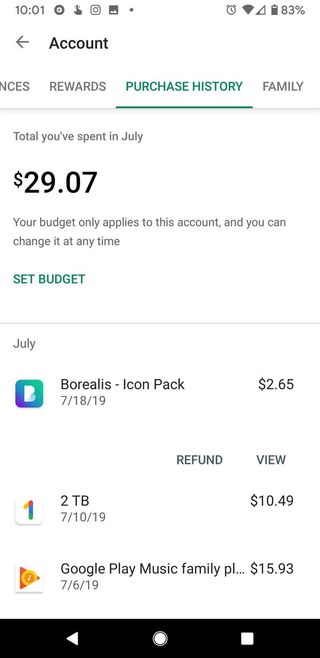The image depicts a smartphone screen with a white background at the top. The status bar displays the time as 10:01 AM. A row of icons follows, including a circle, a finger, the Instagram logo, a PNG label, and a dot. On the right side, there are icons for an alarm clock, Wi-Fi connectivity, 4G signal strength (which is barely filled), and a battery indicator showing 83%.

Below the status bar, on the top-left corner, the word "Account" appears alongside a left-pointing arrow, hinting at a navigation option. Below this, several options are listed, starting with "NCES" (partially visible and cropped from the image), followed by "Rewards," and "Purchase History," which is highlighted in green. "Family" follows next, and a horizontal line separates this section from the next.

The following section reads, "Total You've Spent in July," showing an amount of $29.07. A note indicates, "Your budget only applies to this account, and you can change it at any time," along with a green option button labeled "Set Budget." Below another dividing line, the month "July" is listed, with three entries below:

1. The first entry has a green and purple icon with a paper in the middle, titled "Borealis-iCompact," priced at $2.65, with a date of 7-18-19. Beneath this, options for "Refund" and "View" are shown.
2. The second entry features a white square with a '1' in the middle in Google colors, titled "2TB," priced at $10.49, and dated 7-10-19.
3. The third entry displays a white square with an orange play button, labeled "Google Play Music Family Plan," with a price of $15.93 and a date of 7-6-19.

At the bottom, the image shows the black navigation bar with icons for back (left triangle), home (circle), and recent apps (square).